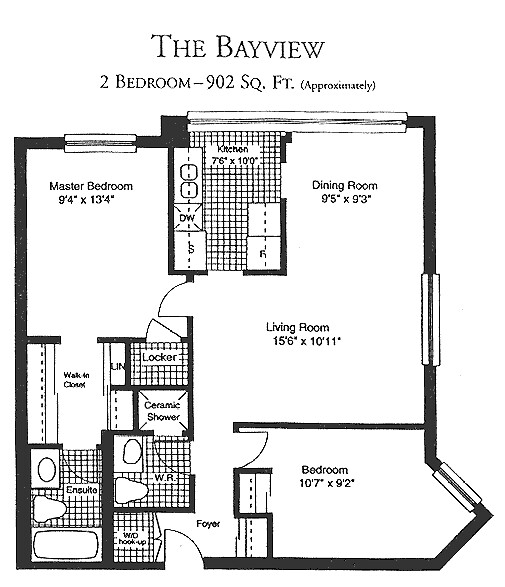This detailed floor plan depicts a 902 square-foot apartment known as "The Bayview." At the top of the layout, it specifies that this is a two-bedroom apartment with an approximate area of 902 square feet.

In the northeast corner of the apartment is the master bedroom, measuring 9 feet 4 inches by 13 feet 4 inches. Adjacent to the southwest of the master bedroom, you'll find a spacious walk-in closet on the west side and a smaller locker to the east. Directly south of the locker, a ceramic shower is situated. The apartment features two bathrooms, each equipped with a toilet and a sink. One bathroom is located south of the walk-in closet, and the other one is positioned to the south of the ceramic shower. In the very southwest corner of the apartment, a bathtub is situated for added convenience.

Centrally located along the northern section of the apartment is the kitchen, which measures 7 feet 6 inches by 10 feet. The kitchen is flanked to the northeast by the dining room, which is 9 feet 5 inches by 9 feet 3 inches. South of the dining room, you will find the living room, which has dimensions of 15 feet 6 inches by 10 feet 11 inches, providing ample space for relaxation and entertainment. Further south of the living room lies the second bedroom, measuring 10 feet 7 inches by 9 feet 2 inches.

The layout provides a well-designed and functional living space, maximizing both comfort and utility.